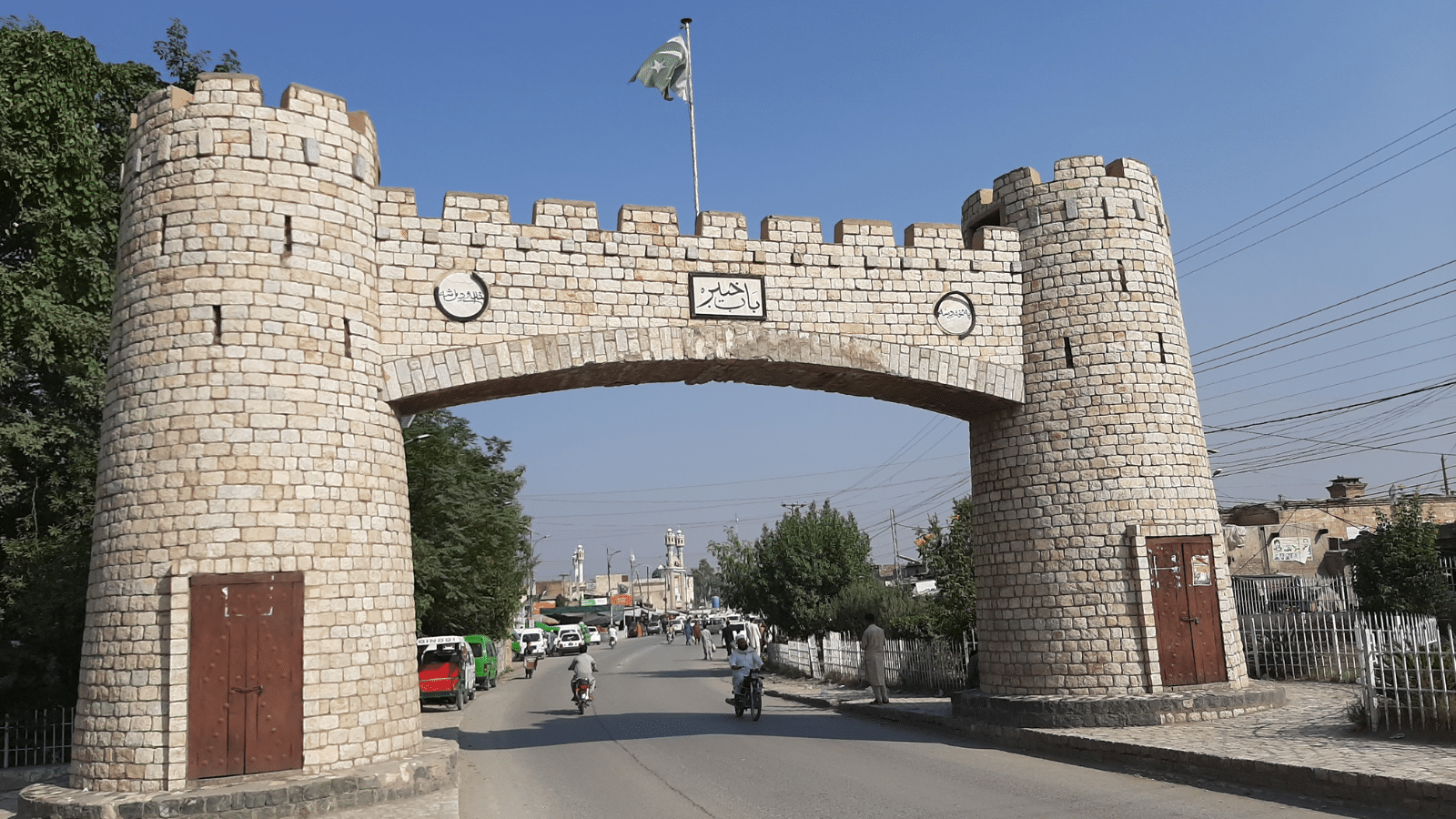The image depicts the entrance of a medieval castle-like structure composed of two cylindrical stone watchtowers. Each tower features brown, wooden double doors at their bases and extends upward to crenellated parapets, which provide protection for guards while offering vantage points. The two towers are connected by a rectangular stone bridge that arches slightly at the bottom, mirroring the watchtowers' crenellated design. A white flag ripples from a flagpole at the center of the bridge. Below the bridge, which spans a street, small colorful cars (white, red, and green) are parked alongside a few motorcycles or mopeds driving away from the viewer. The scene is set against a light blue sky, free of clouds, and flanked by lush green trees on the left and telephone or electrical lines on the right. In the background, more buildings, possibly cathedrals or mosques, hint at a bustling cityscape not far from this picturesque castle gate.